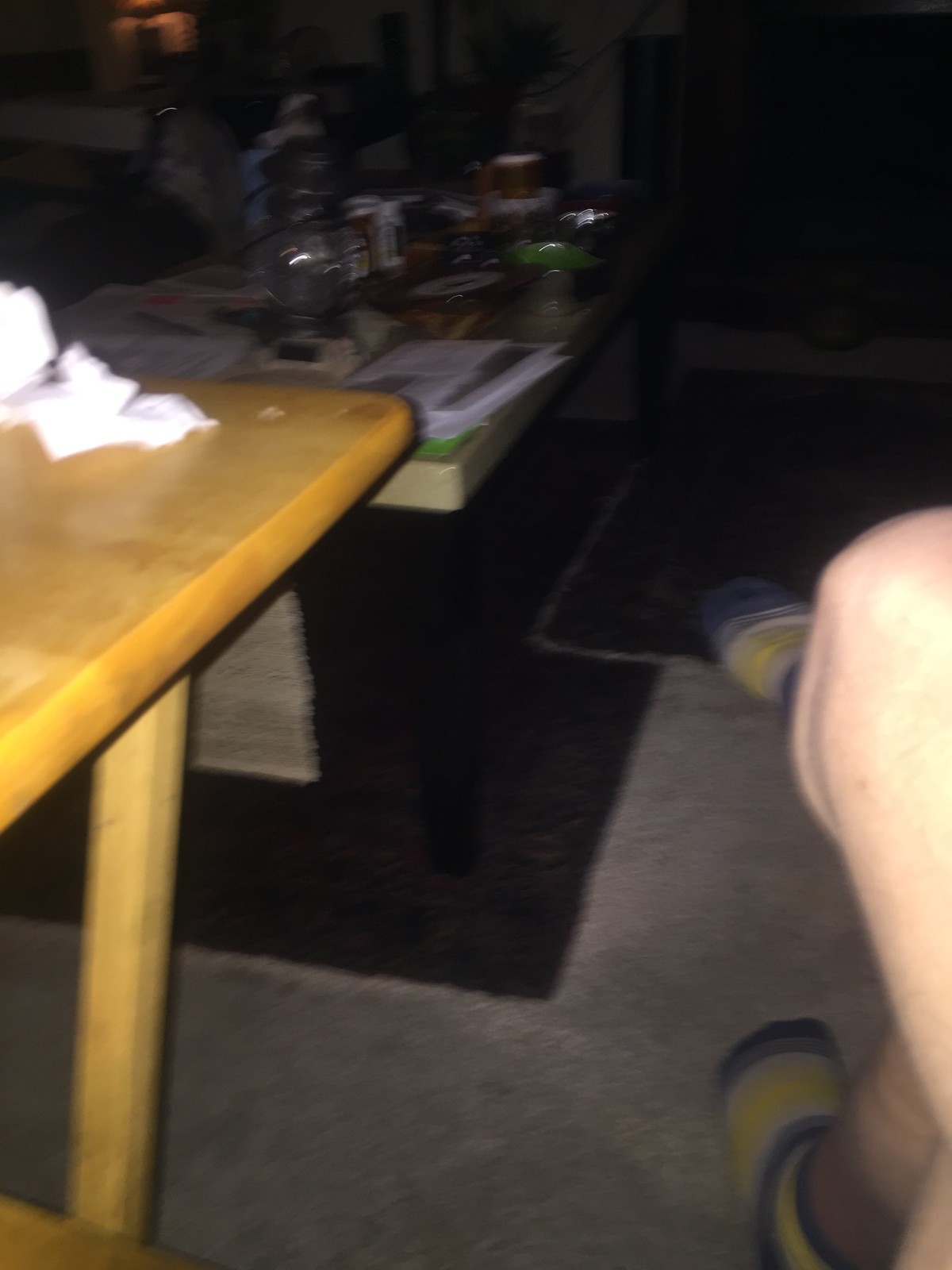In the photograph, the focal point is on the right side, where a person's bare legs are visible, adorned only with colorful striped socks in dark blue, light blue, white, and yellow. The individual is positioned in such a way that we cannot see any more of their body. On the left side of the image stands a wooden table, likely a TV table given the angled legs suggesting it may be foldable. The room beyond is shrouded in darkness, making it difficult to discern details. There are, however, some papers and possibly a book resting on a black surface, with some indistinct reflections visible in the background, adding a mysterious ambiance to the scene.